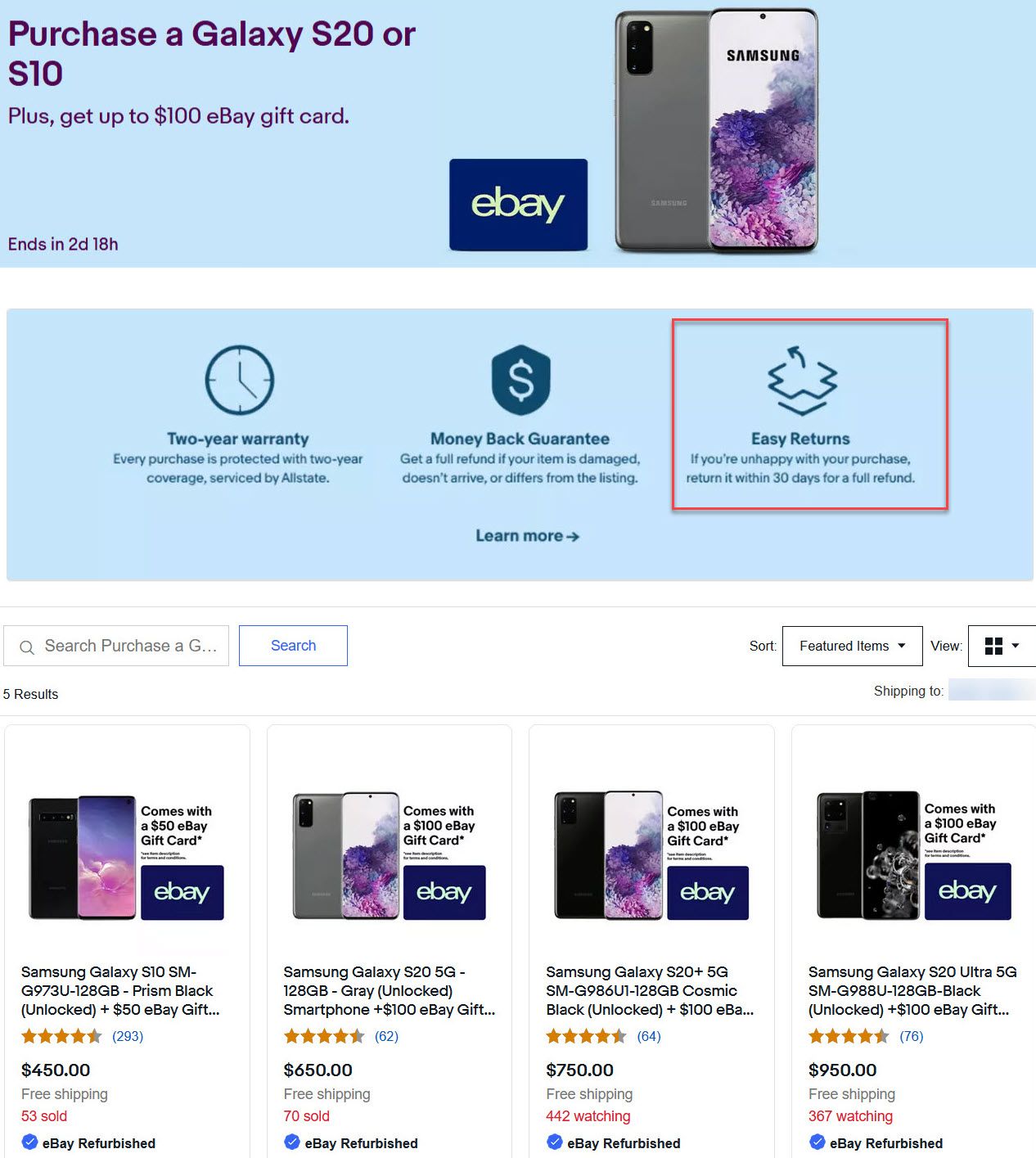This is a screenshot taken from a device, likely a phone or computer, showcasing an eBay promotional page. At the top, there are two blue rectangles. The first blue rectangle contains a promotional offer that reads, "Purchase a Galaxy S20 or S10," followed by smaller text stating, "plus get up to $100 eBay gift card." In the left-hand corner of this rectangle, in very small print, it notes, "ends in two days 18 hours." Immediately below, within a navy rectangle, is the eBay logo.

The central part of the image highlights the back of a cell phone, which appears to be in a chrome color, showcasing its camera area prominently. The phone is powered on, displaying the Samsung logo against a white background accented with purple, blue, and pink hues.

Further down the page, another rectangle features icons and text: a clock symbol accompanied by "Two-Year Warranty," a shield emblem with an "S" denoting "Money Back Guarantee," and finally, a red-bordered section that says "Easy Returns."

The bottom portion of the screenshot displays four different buying options, each with star ratings visible, providing detailed options for prospective buyers.